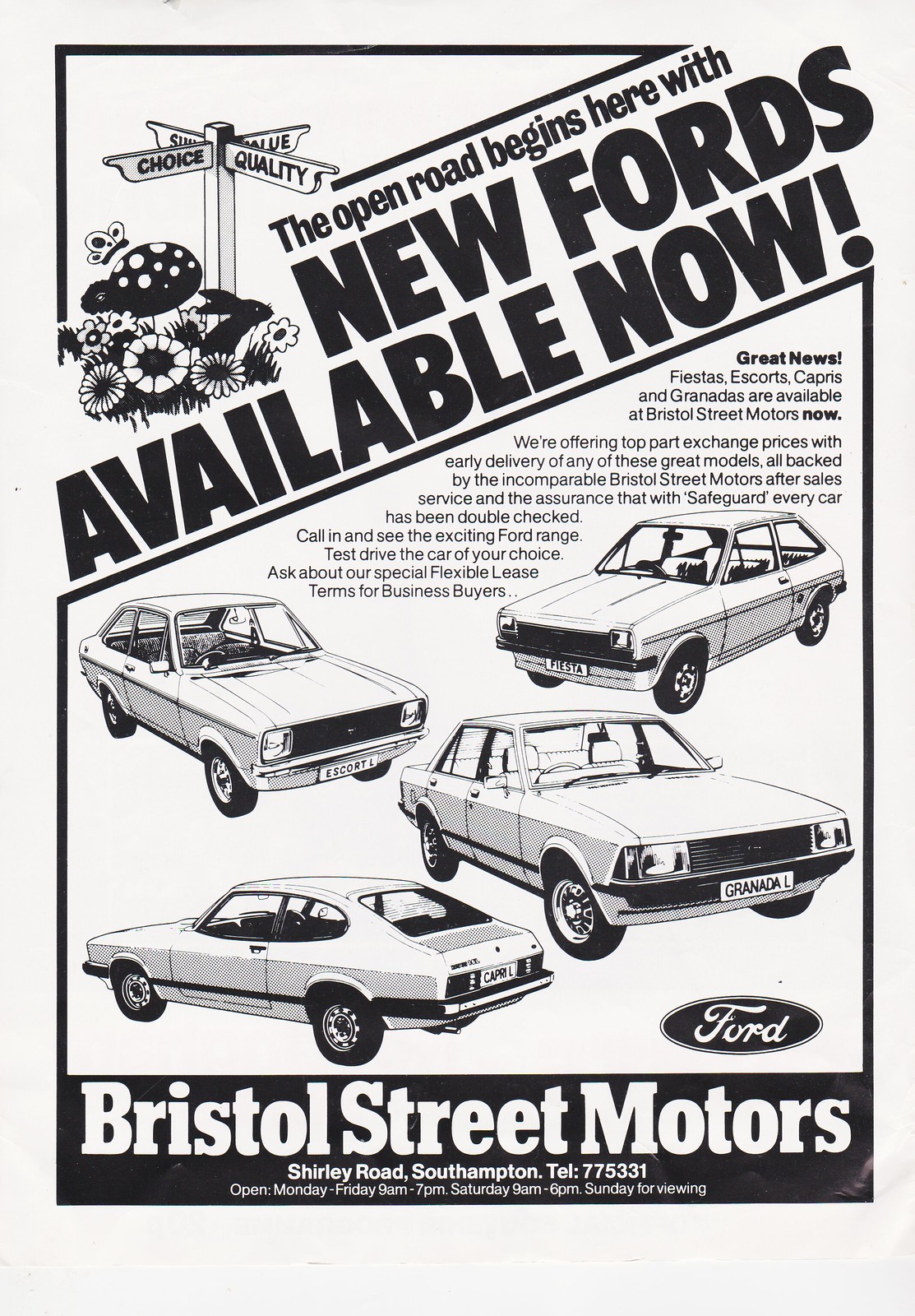This vertically aligned rectangular image is an old advertisement with a light gray or white background typical of aged newspaper. Across the top, it reads in a smaller black font, "The open road begins here with," followed by a bold, diagonal title in all caps, "NEW FORDS AVAILABLE NOW!" In the upper left-hand corner, there is an image of a street sign with words like "Choice" and "Quality" and intricate details of flowers and butterflies below it. The middle section of the ad prominently features images of five different Ford cars, possibly from the 1960s, accompanied by right-aligned text. The lower right-hand corner displays the iconic Ford logo. At the very bottom, bold white letters announce "Bristol Street Motors," with the address, "Shirley Road, Southampton, telephone 775-331," and operating hours: Monday through Friday from 9 a.m. to 7 p.m., Saturday from 9 a.m. to 6 p.m., and Sunday for viewing. The entire ad is outlined with a black border.